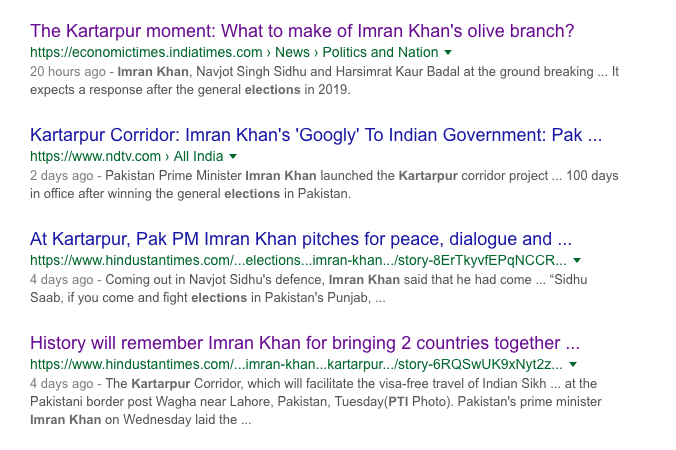The image depicts a series of search results reminiscent of a Google search page. The top result, highlighted in purple, reads, "The Kartarpur Moment: What to Make of Imran Khan's Olive Branch?" This suggests an article focused on the diplomatic efforts of Imran Khan concerning the Kartarpur Corridor. Below this, there is a clickable link from the website "economictimes.indiatimes.com," marked with a timestamp indicating it was posted 20 hours ago.

The second search result is in blue and says, "Kartarpur Corridor: Imran Khan's 'Googly' to Indian Government." This title suggests a complex or surprising move by Imran Khan, likened to a deceptive delivery in cricket.

The third search result reads, "At Kartarpur, Pak PM Imran Khan Pitches for Peace, Dialogue, and..." The ellipsis indicates additional, perhaps significant, information following the truncated title.

The fourth and final search result, also in purple, states, "History Will Remember Imran Khan for Bringing Two Countries Together." This likely reflects a positive perspective on Khan's efforts to foster peace.

The last text in green is from the "www.hindustantimes.com," starting with "imran-khan," followed by an ellipsis and "kartarpur-ellipses-story.” This article was posted four days ago, indicating a relatively recent development.